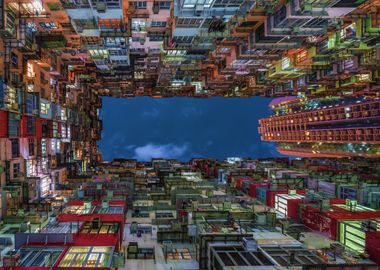The image depicts a highly detailed, possibly computer-generated view of a densely built urban courtyard taken from a low-angle perspective. The scene showcases towering buildings, reminiscent of skyscrapers with multiple floors, balconies, and numerous windows. These buildings vary in color, including red, gray, pink, blue, and more, and many of the windows emit light, adding a vibrant diversity to the night setting. The center of the image features a rectangular blue area that appears to be a pool. Additionally, the right-hand side of the image includes a uniquely shaped, possibly circular structure, enhancing the scene's eclectic architectural mix. The overall impression is one of a bustling, vividly lit cityscape observed from a novel vantage point.